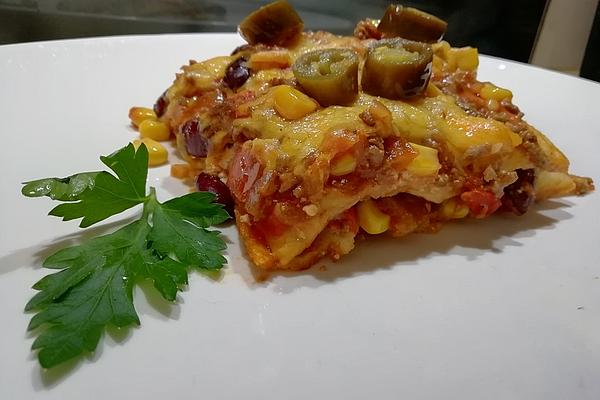The image depicts a high-quality photograph of a layered entree, resembling lasagna, presented on a circular white plate. This square-shaped dish features several distinct layers and ingredients. On top, there are thickly sliced, pickled jalapenos, under which lies a generous layer of melted cheese. Beneath the cheese, a layer of red sauce is visible, complemented by scattered corn kernels. Further down, there is a layer that appears to be either pasta or a tortilla, followed by additional sauce and corn. To the left side of the entree, a sprig of green herb, possibly cilantro or parsley, adds a fresh touch. The background of the photo shows a slight reflection, suggesting the presence of a window in the scene. The dish is carefully plated on a white plate, which rests on a table, ready to be enjoyed.